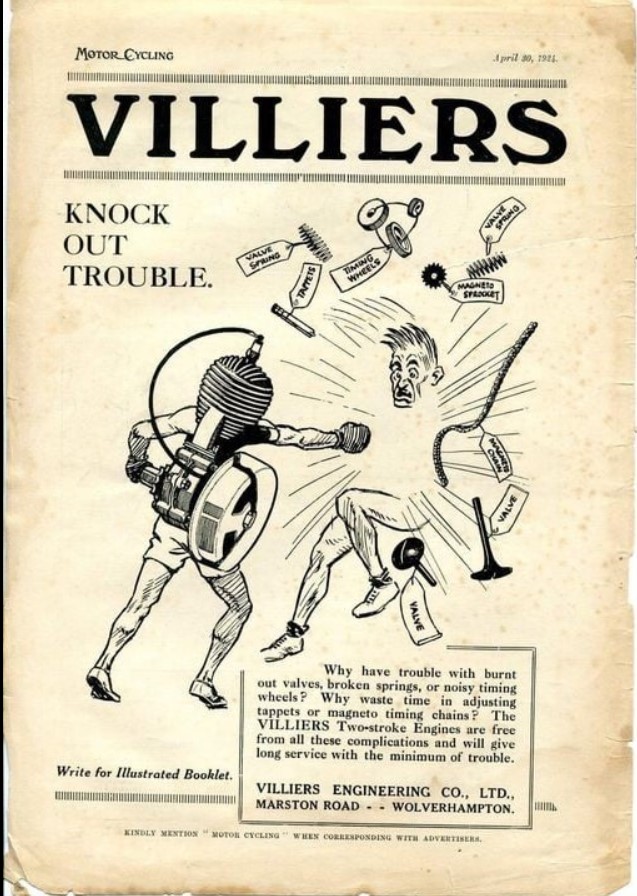This photograph captures the cover of an old pamphlet or magazine dated April 20th, 1921, prominently featuring the title "Motor Cycling" in the upper left corner. Beneath this, the name "Villiers" is emblazoned in large black letters followed by the headline "Knockout Trouble." The focal illustration depicts a dramatic and somewhat cartoonish scene where a machine-like figure with legs and a spark plug on its head, wielding a flywheel on its right, is forcefully punching a man. The impact has caused various motor parts, including a hammer, valve, springs, and other metal objects, to scatter through the air. Accompanying this scene is a detailed promotional text inside a square at the bottom, which reads: "Why have trouble with burnt out valves, broken springs, or noisy timing wheels? Why waste time in adjusting tappets or magneto timing chains? The Villiers two-stroke engines are free from all these complications and will give you long service with the minimum of trouble." At the very bottom, it lists "Villiers Engineering Company, Marston Road, Wolverhampton." The cover’s background is a light pink, while all the printed text is in black, creating a stark contrast that draws attention to the advertisement's message.